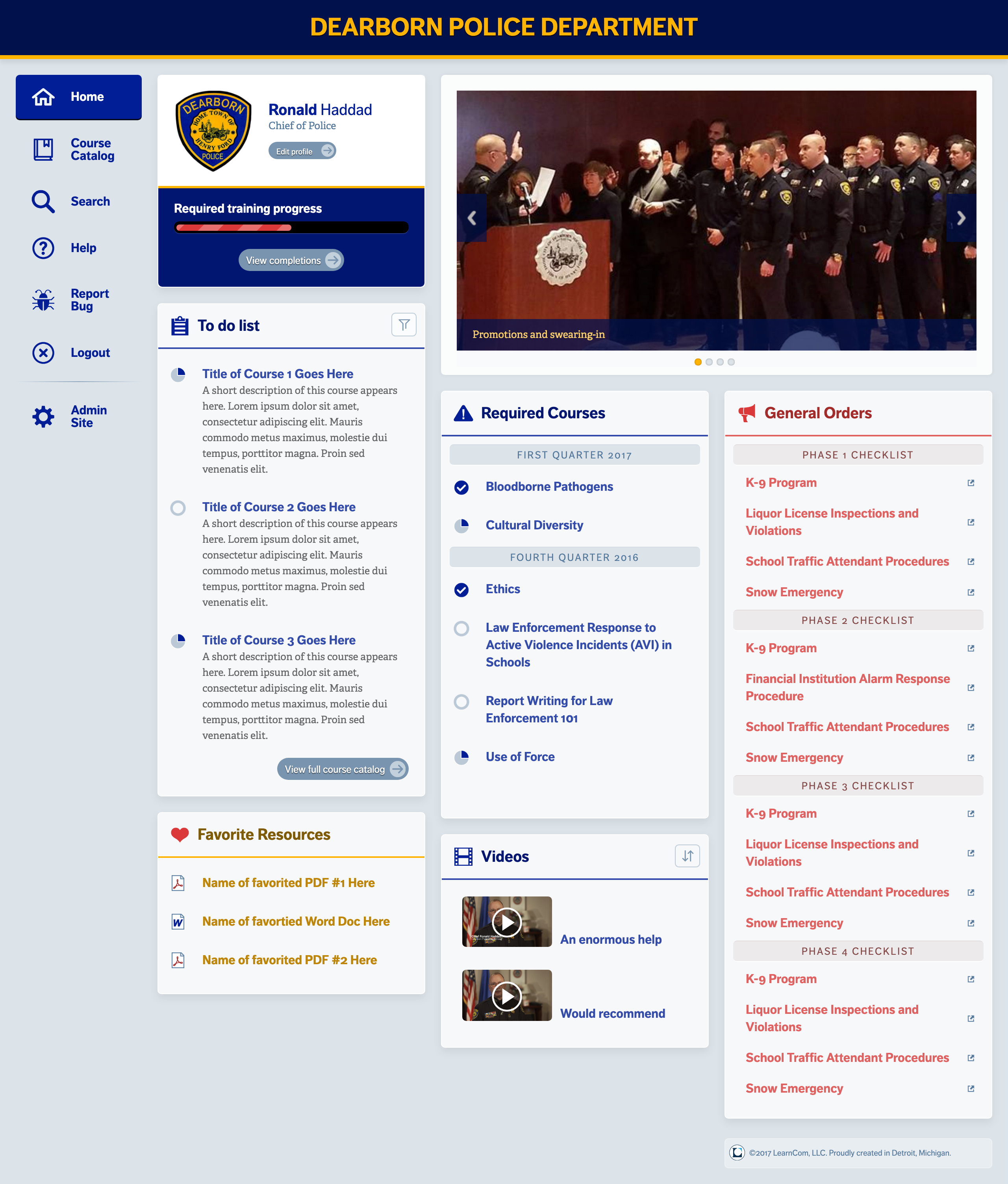This is a web page for the Dearborn Police Department. The page prominently features the following tabs: Home, Course Catalog, Search, Court Bug, Law Gown, and Admin Site. It clearly states Ronald Haddad as the Chief of Police. The main section of the page is dedicated to ongoing training, labeled "Acquired Training in Progress." Below this, there's a listing area titled "Title of Course," which has placeholders for multiple course names.

Additionally, the page includes a detailed to-do list outlining required courses, such as "Bloodborne Pathogens," "Cultural Diversity," "Ethics," and "Law Enforcement Response to various situations." There is a comprehensive checklist categorized into phases: Phase 1, Phase 2, Phase 3, and Phase 4. Alongside these phases are listed resources needed for the training and completion of these courses. The webpage seems to serve as a reporting tool for individuals undergoing the training program.